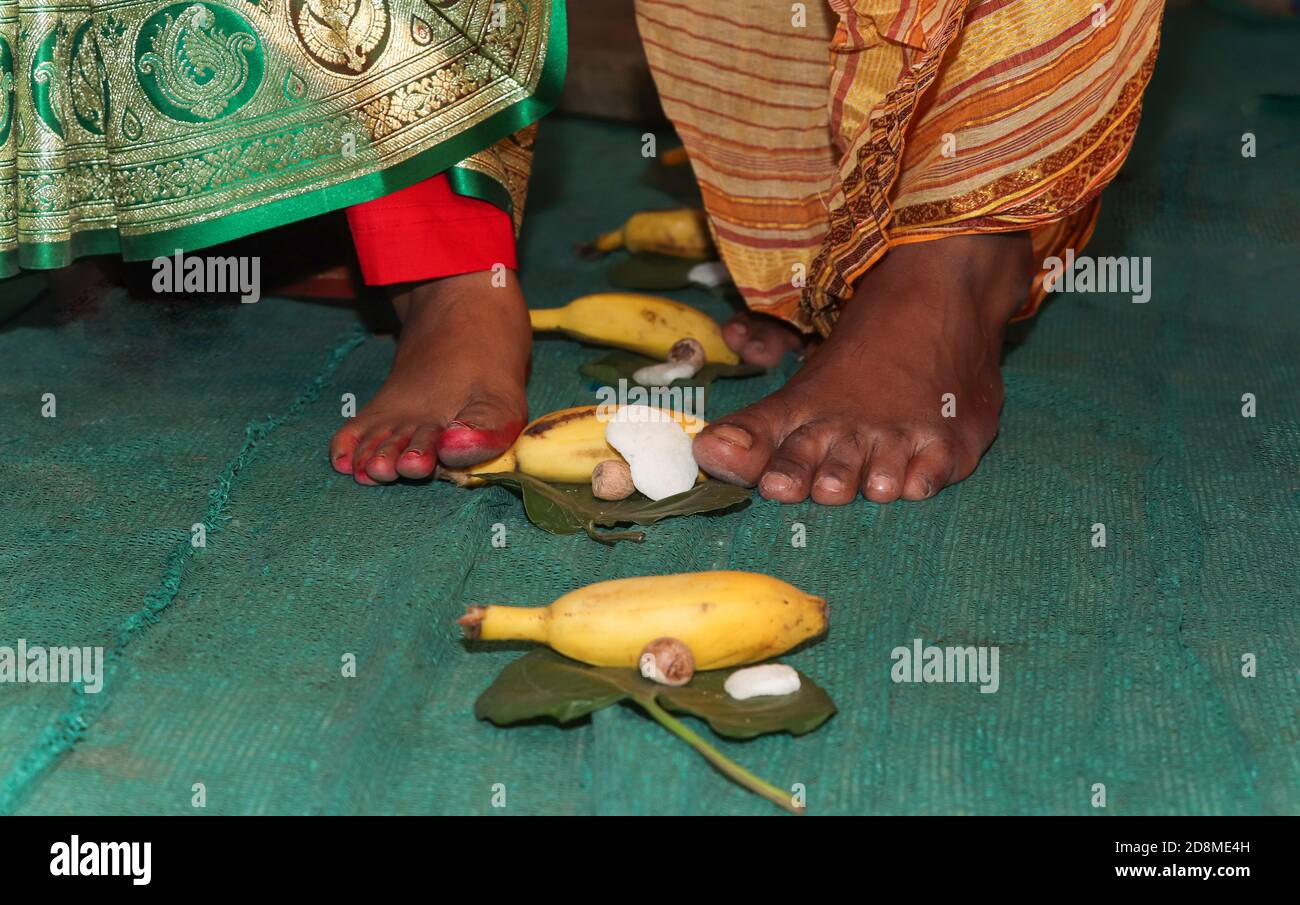In the image, there is a close-up shot of a person's bare toes positioned on top of a fabric. The individual is barefoot and standing in front of others, with a fabric surface beneath their feet. Interspersed between their legs is a nest adorned with green leaves, arranged in an upward line. Each leaf bears a banana and a peanut, along with some small white objects. The person is dressed in a red trouser, with an additional piece of fabric draped above it, showcasing a pattern of yellow, brown, green, and gold.

The photograph is overlaid with several green watermarks that read "Alami," prominently featured five times in the center. Additional 'A's are scattered across the image as part of the watermark pattern. At the bottom of the image, there is a black header bar. On the bottom left of this bar, "Alami" is written in white text. On the bottom right, there is white text that reads "Image ID 2D8ME4H" along with the website "www.alami.com." 

The overall image appears marked by these numerous gray watermarks and has a specific, detailed layout that emphasizes the feet, the fabric, and the arranged leaves with bananas and peanuts.